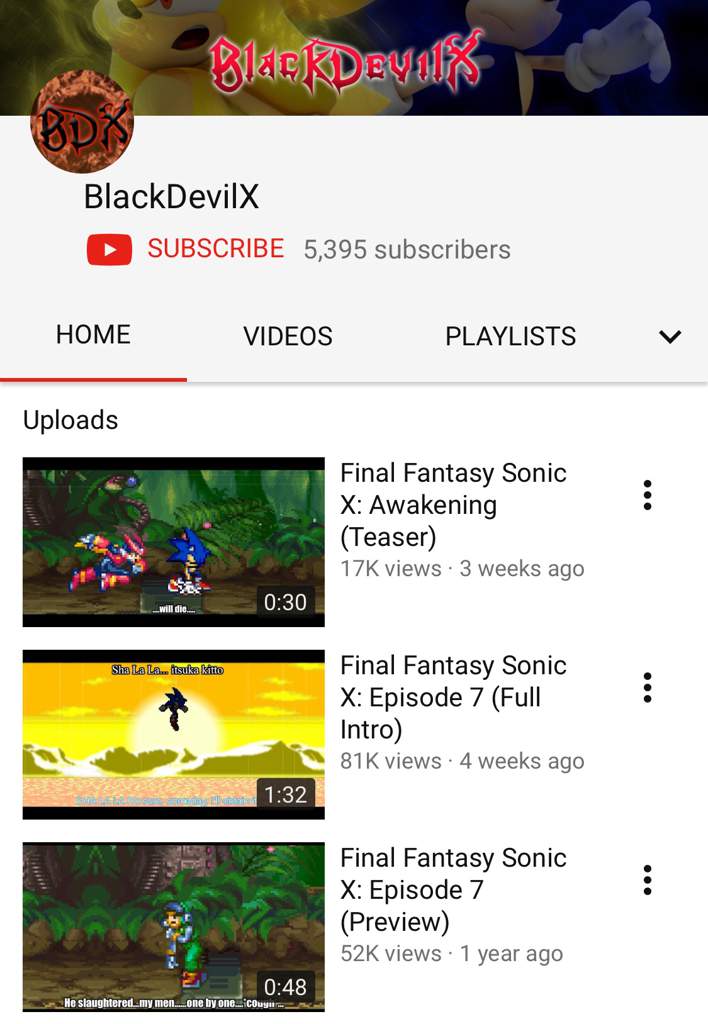The image features a white background with a header section at the top. The header contains a small, dark green and blue picture with a little yellow character. The text "Black Devilix" appears in red letters. Adjacent to this image, there is a small circle with a reddish image that has "BDX" written on it. Below this, the text "Black Devil X" appears along with a red rectangular button containing a white right arrow and the word "Subscribe" in red text. The subscriber count reads "5,395 subscribers".

Below the header, there are navigation links with the word "Home" underlined with a red line, followed by "Videos", "Playlist", and a down arrow. The section below the navigation links has a title "Uploads" set against a white background. Under "Uploads," there are three listed video thumbnails:

1. The first video is titled "Final Fantasy Sonic X Awakening Teaser" and has 17,000 views, posted three weeks ago, with three little dots on the right for additional options.
2. The second video titled "Final Fantasy Sonic X Episode 7 Full Intro" has 81,000 views, posted four weeks ago, also with three dots on the right.
3. The third video is "Final Fantasy Sonic X Episode 7 Preview" with 52,000 views, posted one year ago, accompanied by the same three-dot menu on the right.